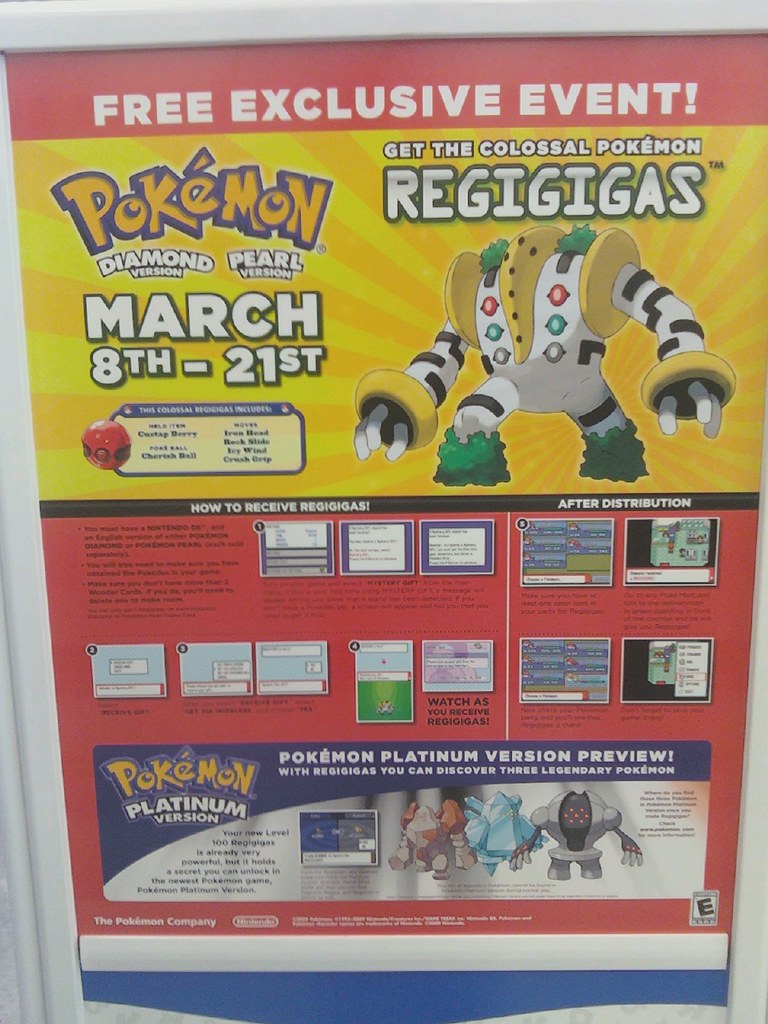The poster is for a Pokémon event and is prominently displayed in another language. At the top, a bold red banner screams "FREE EXCLUSIVE EVENT" in all caps, highlighted by an exclamation point below it. The iconic Pokémon logo in vivid yellow is positioned right beneath the banner. Below the logo, two different game versions are mentioned: "Diamond Version" and "Pearl Version," with the "Diamond Version" text stylishly curved.

The event dates, March 8th to 21st, are clearly stated underneath. Dominating the center of the poster is an eye-catching image of Regigigas, one of the Colossal Pokémon. Regigigas is depicted with green moss-like legs and shoulders, white and black-striped arms, and yellow rings around its shoulders and wrists. 

To the left of Regigigas is a section detailing how to receive specific items, labeled "This Colossal." If you purchase the indicated toy, various items can be received, and a step-by-step guide is provided. This guide consists of four steps, followed by four snapshots each with descriptions that explain the process.

Near the bottom of the poster, there's a mention of the "Pokémon Platinum Version," accompanied by images illustrating different aspects of the game. The event is sponsored by Nintendo, and the poster features the "E for Everyone" rating logo at the bottom.